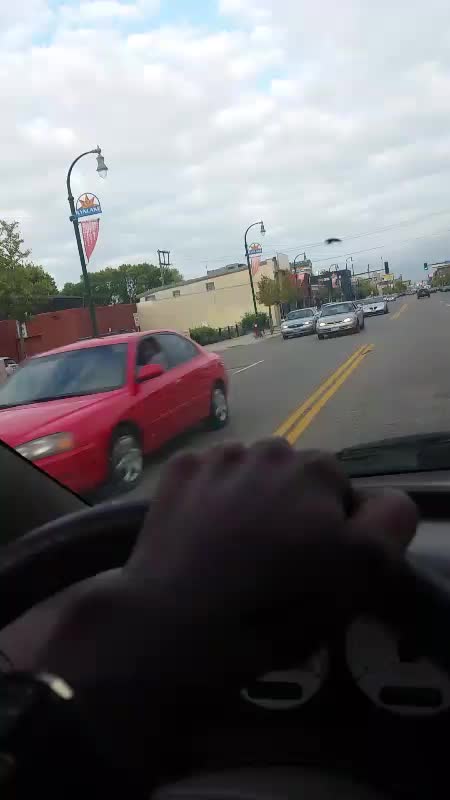A view from the driver's seat in an African-American man's car reveals his hand, adorned with a watch, gripping the steering wheel. The scene outside the windshield depicts a dreary day on a two-lane road, both lanes heading in each direction. Street lights line the road, many of them displaying flags, though the inscriptions are unclear. In the left-hand lane, close to the double yellow lines, the driver is passed by a red car, while two to three gray cars approach from the opposite direction. In the distance, a green traffic light stands, offering a chance to proceed without stopping.